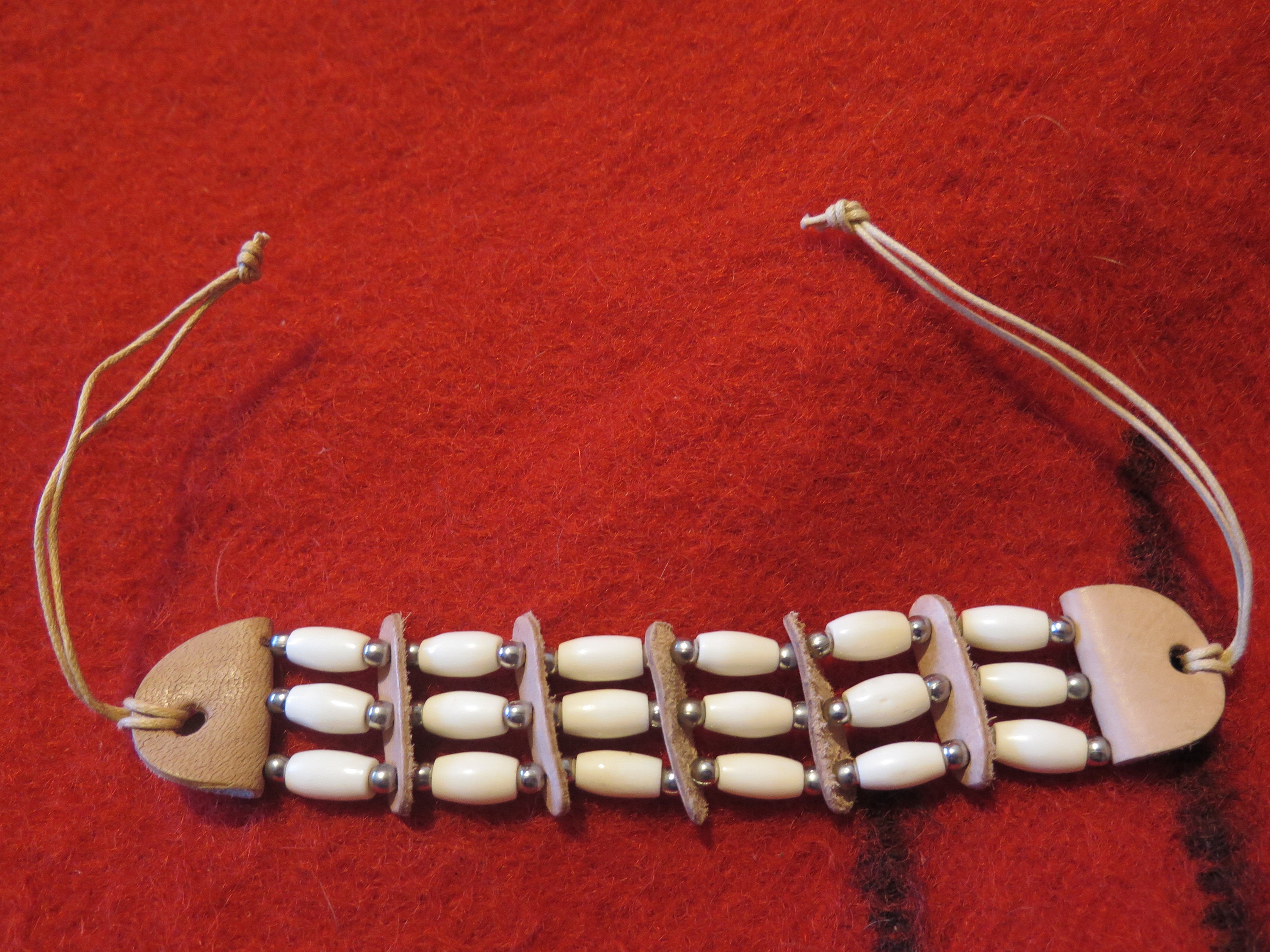The image depicts a handcrafted bracelet elegantly laid on a vivid red wool blanket adorned with a few black stripes. The intricate bracelet, which stands out starkly against the bright backdrop, features tan leather ties on each end, designed to be fastened around the wrist. The centerpiece of the bracelet consists of six rows of cylindrical white beads, each bead capped with tiny silver balls. Between each row of beads are slender pieces of leather, providing both structure and aesthetic separation. The bracelet showcases an alternating pattern of beads and leather dividers, except for the sixth row, which directly connects to the leather ends. The bright and textured red blanket, with its black lines radiating from the bottom right, enhances the artisanal beauty of the bracelet.